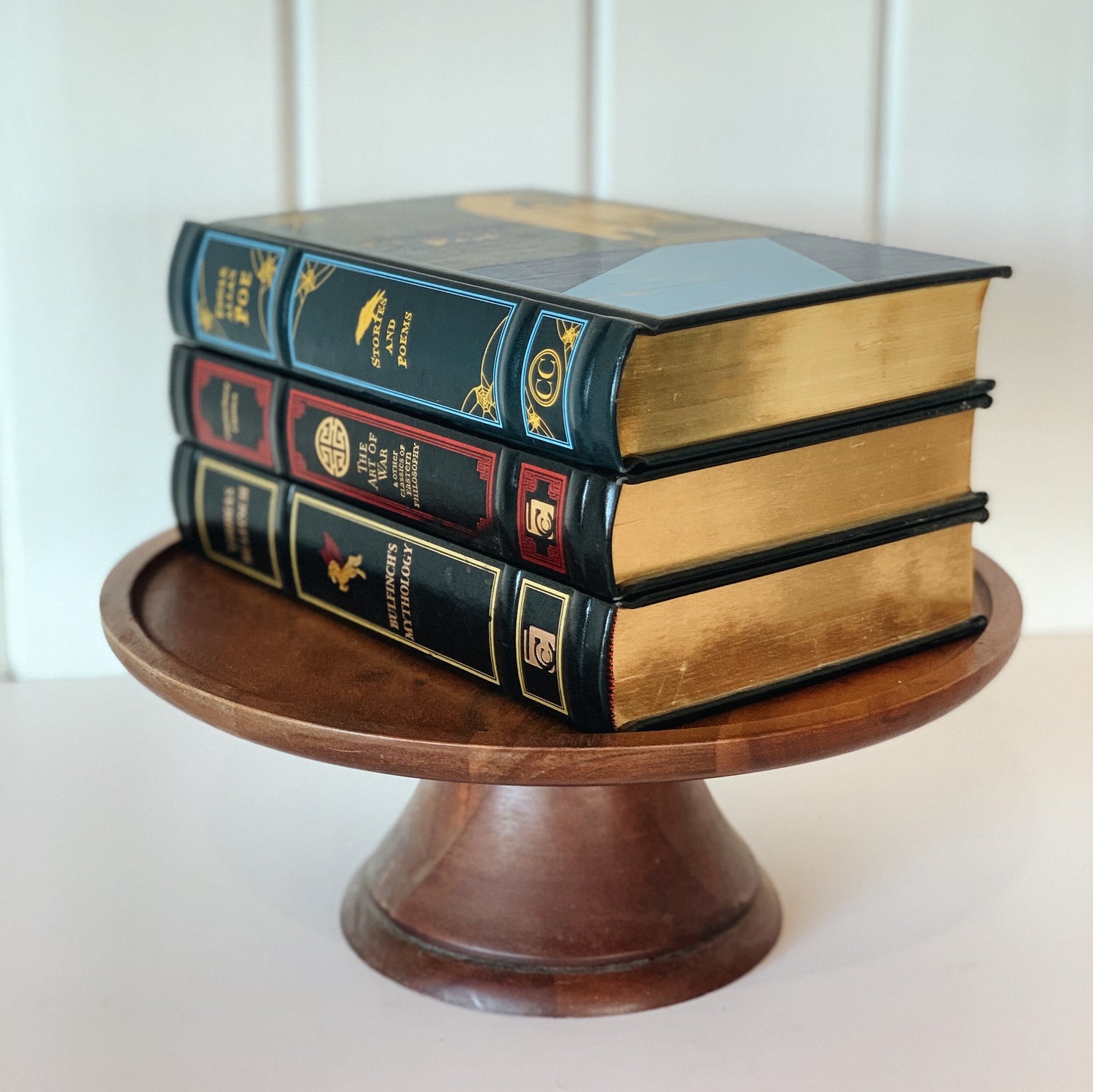This detailed color photograph features a stack of three hardcover books, elegantly arranged on a polished, round wooden pedestal with a tapered, darker base. The pedestal is placed against a backdrop of white wooden panels, creating a striking contrast. Each book is predominantly black with gold-gilded page edges that shimmer softly in the light.

The topmost book, adorned with blue and yellow decorations, reads "Short Stories and Poems" and appears to be authored by Edgar Allan Poe, though the text is slightly blurred. The middle book, highlighted with red patterns, is identifiable as "The Art of War." The bottom book, with silver text and illustrations of a red and gold Pegasus, is titled "Bullfinch's Mythology."

The wooden pedestal itself features a shallow, carved indentation, perfectly accommodating the books. The overall setting, possibly on a beige shelf or table, adds to the image's refined and scholarly ambiance.